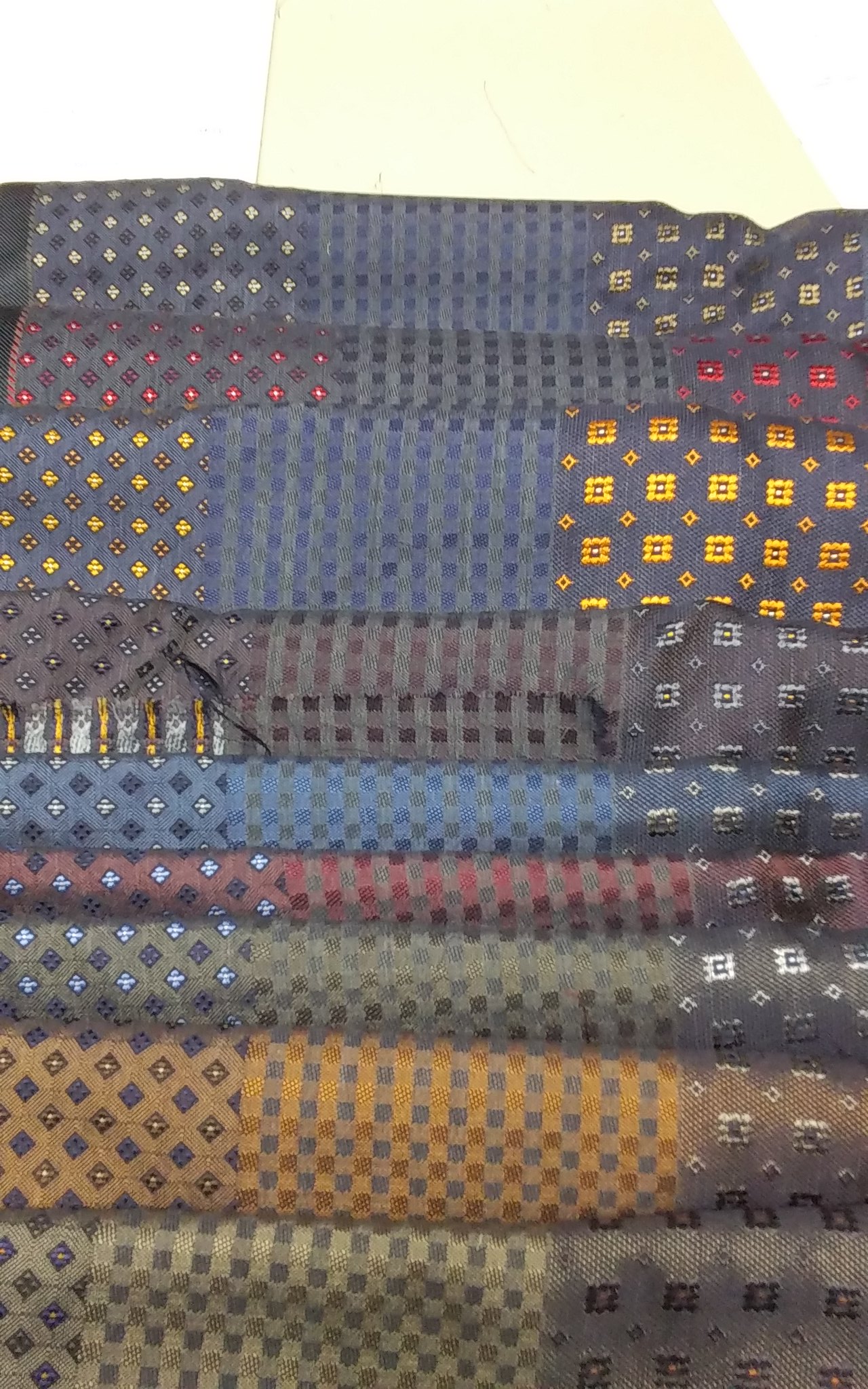This color photograph captures a neatly stacked array of various fabrics, each folded and arranged both vertically and horizontally. The textures of the fabrics are shiny and fine, reminiscent of the material used to make neckties, foulards, or pocket squares. The fabrics display small, elegant, masculine patterns, including diamonds, squares, lozenges, and star motifs. The predominant hues in the photograph are somber and muted, featuring dullish blues, browns, and a brownish-green, with accents of orange, red, gray, black, and a touch of yellow. The fabrics are stacked in approximately ten visible layers, set against a white backdrop with a pale yellow tint at the top.